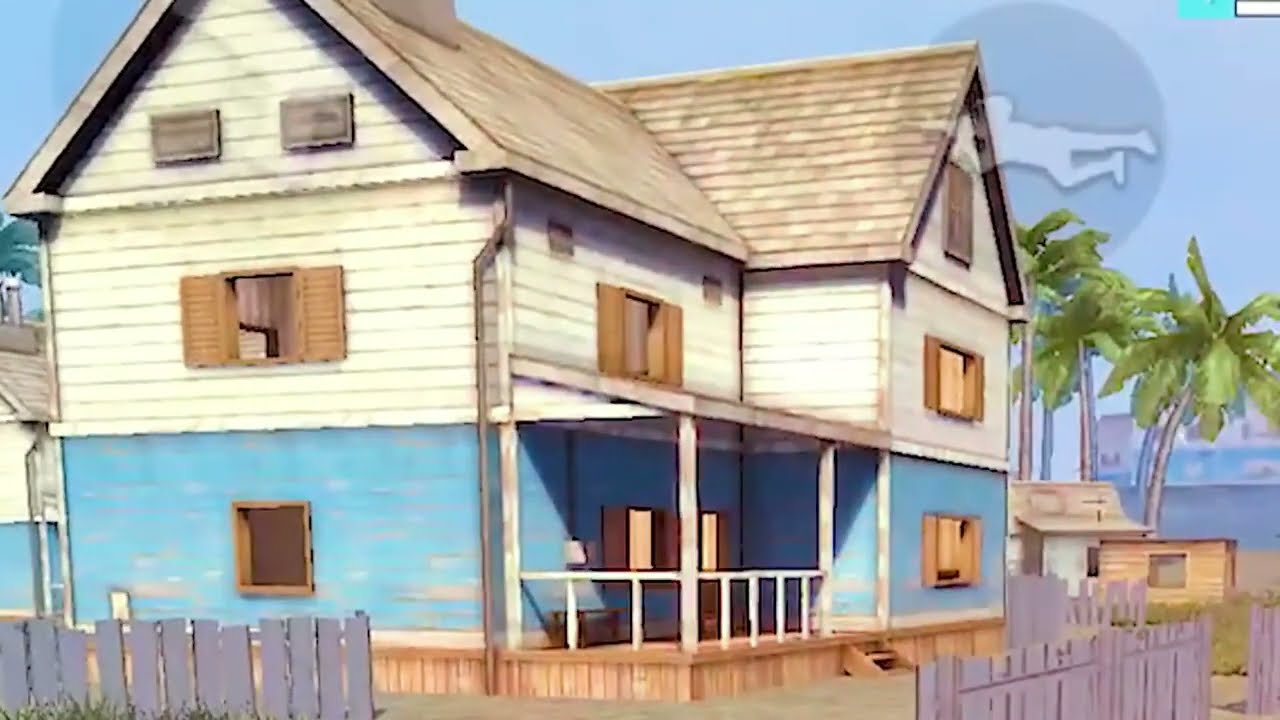The image is a detailed and digitally rendered scene, likely from a video game or as an artwork with a watercolor or filtered aesthetic. The central focus is a three-story house, with the bottom half featuring blue paneled walls and the top half in white. The light brown roof caps the structure, complemented by brown windows with open wooden shutters. A wooden front porch with pillars and rails adds to the house's quaint charm, anchored by a brown wood foundation.

Surrounding the house, light grayish-brown and gray fence posts define the yard's boundaries, with entrances at the bottom left and right corners. To the right of the house, several lush palm trees with light brown trunks stand tall, and beneath them are smaller, one-story wooden houses and huts. The scene is bathed in hues of light blue, light purple, gray, green, dark green, beige, brown, white, black, and tan, creating a vibrant and layered visual experience.

Adding a surreal touch, a shadowy silhouette of a child appears to be floating into the house from the top right corner, enhancing the mysterious and artistic quality of the image. The overall style evokes a mix of digital art and filtered photography, capturing an intriguing, whimsical atmosphere.